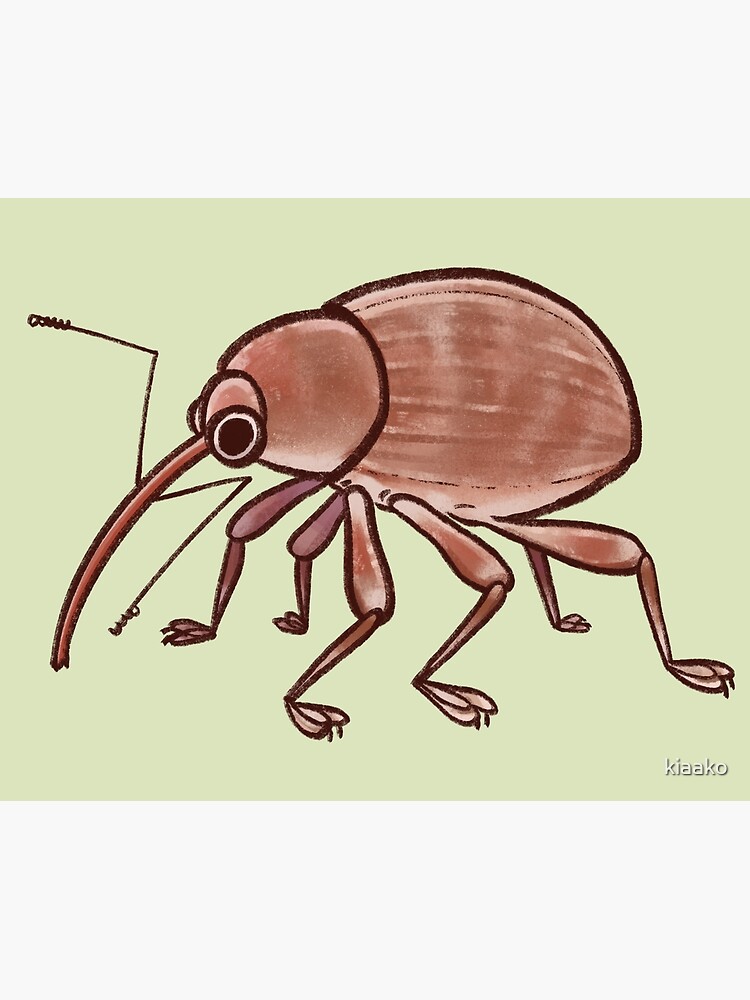The image is a detailed, colored cartoon drawing of a bug, most likely a flea, centered on light gray or tan paper. The bug, facing left, showcases a round, pecan-like body and a smaller, roundish head with large white eyes. A notable feature is its elongated, narrow proboscis that extends from the front of its head, touching the ground, suggesting it may be used for feeding. The insect has two antennae, about a third of the way down from its head, forming zigzag patterns with small fuzzy zigzags perpendicular to the main lines. It is equipped with six legs, each ending in three toes, with the center toe resting above the others. The visually striking black writing at the top left continues in a line that wraps behind the proboscis and under the right eye, joining more text in front of the bug's right front leg. Additional white writing is visible in the bottom right-hand corner, beside the word "kiako."